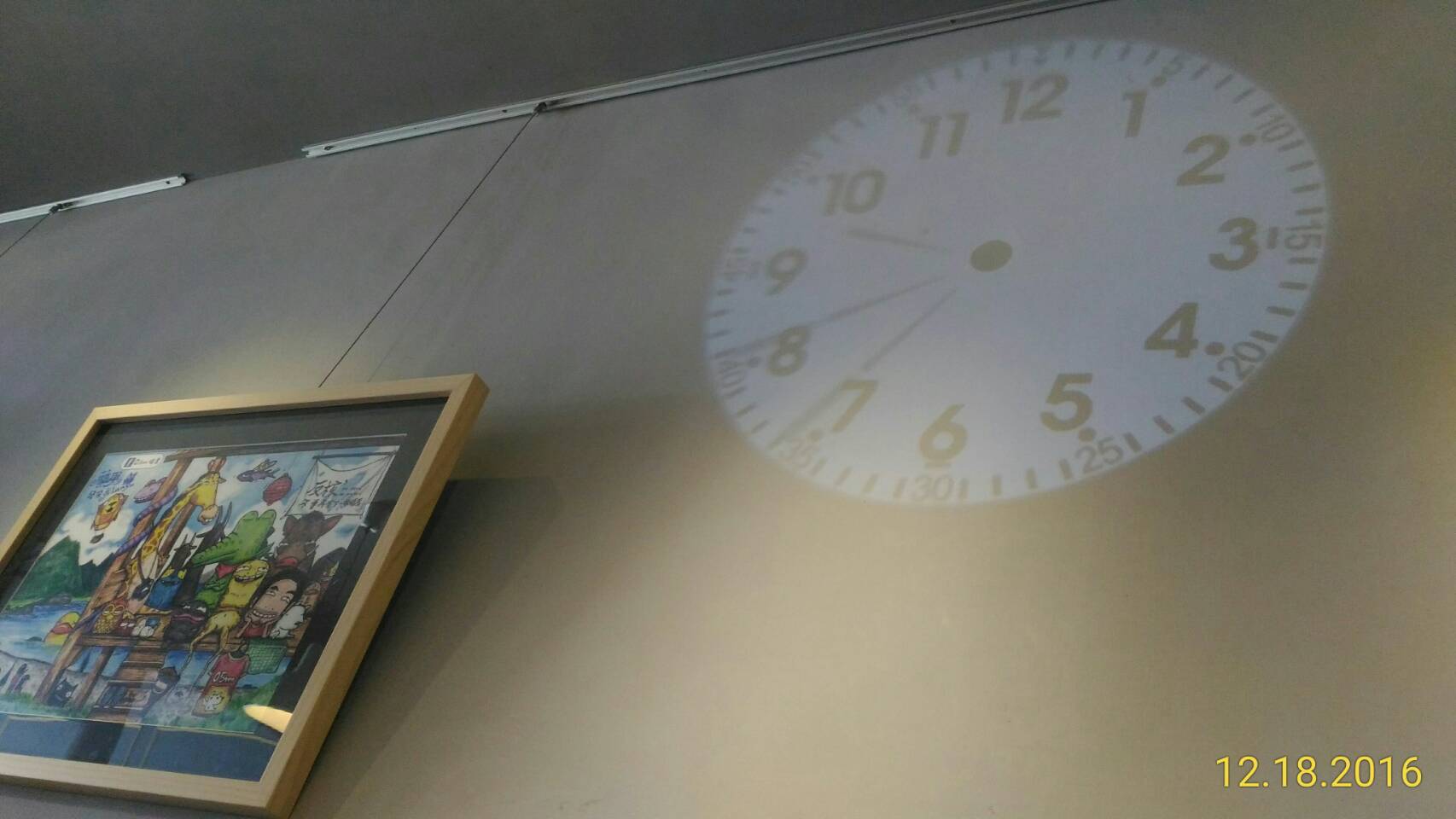The image features a gray wall with a distinctive focal point on the top right: a clock or a clock-like face possibly painted directly onto the wall. The clock face is white with black numerical markings and minute indicators. A series of dark lines are visible on the clock face, particularly around the numbers 7, 8, and a smaller line near 10. The center of the clock is black. To the left and slightly below the clock, there is a picture hanging on the wall in a brown frame. The picture depicts a group of colorful cartoon characters standing together. The ceiling, visible in the image, is a darker shade of gray compared to the wall. In the bottom right corner, there is a timestamp reading "12.18.2016".